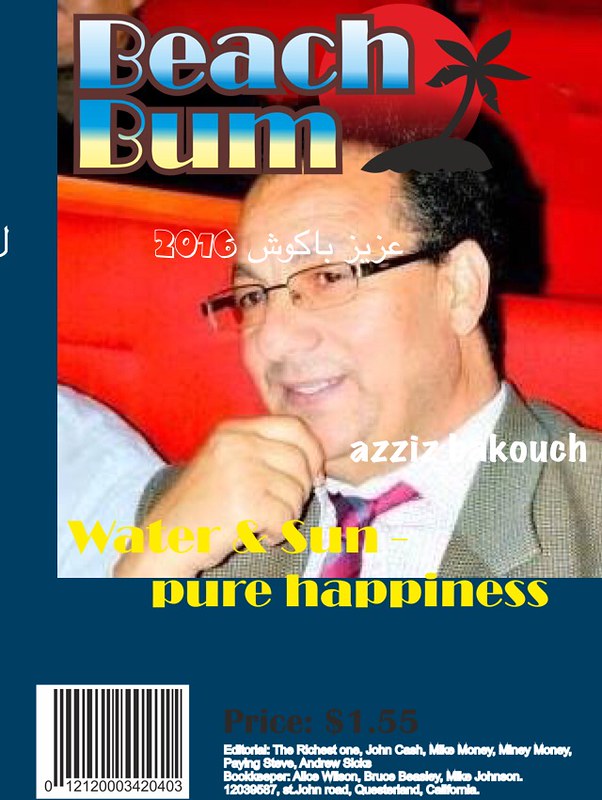The magazine cover predominantly features a dark blue background, with a prominently placed vertical rectangle photo occupying about two-thirds of the cover's center. The photo showcases an older man, around 50 years old, with tan skin, balding but having black and gray hair on the sides. He wears rectangular black glasses with thin fronts and thick outer borders. Dressed in a gray suit with a white shirt and a purple tie, he is seated in a red chair, leaning slightly and resting his right fist under his chin. Above his head, in thick stylized letters with a brown outline and a blue-to-white gradient fill, the headline "Beach Bum" is prominently displayed. To the right of the headline, there is a black icon of a palm tree, and beneath it, the year "2016" is printed. Some foreign font (possibly Arabic) and the name "Aziz Bakuch" are written in white across his collar, although partially obscured. At the bottom, yellow text reads, "Water and Sun: Pure Happiness." Pricing information is noted in black with "$1.55" and additional editorial text and numbers, including a barcode, are located toward the bottom left.